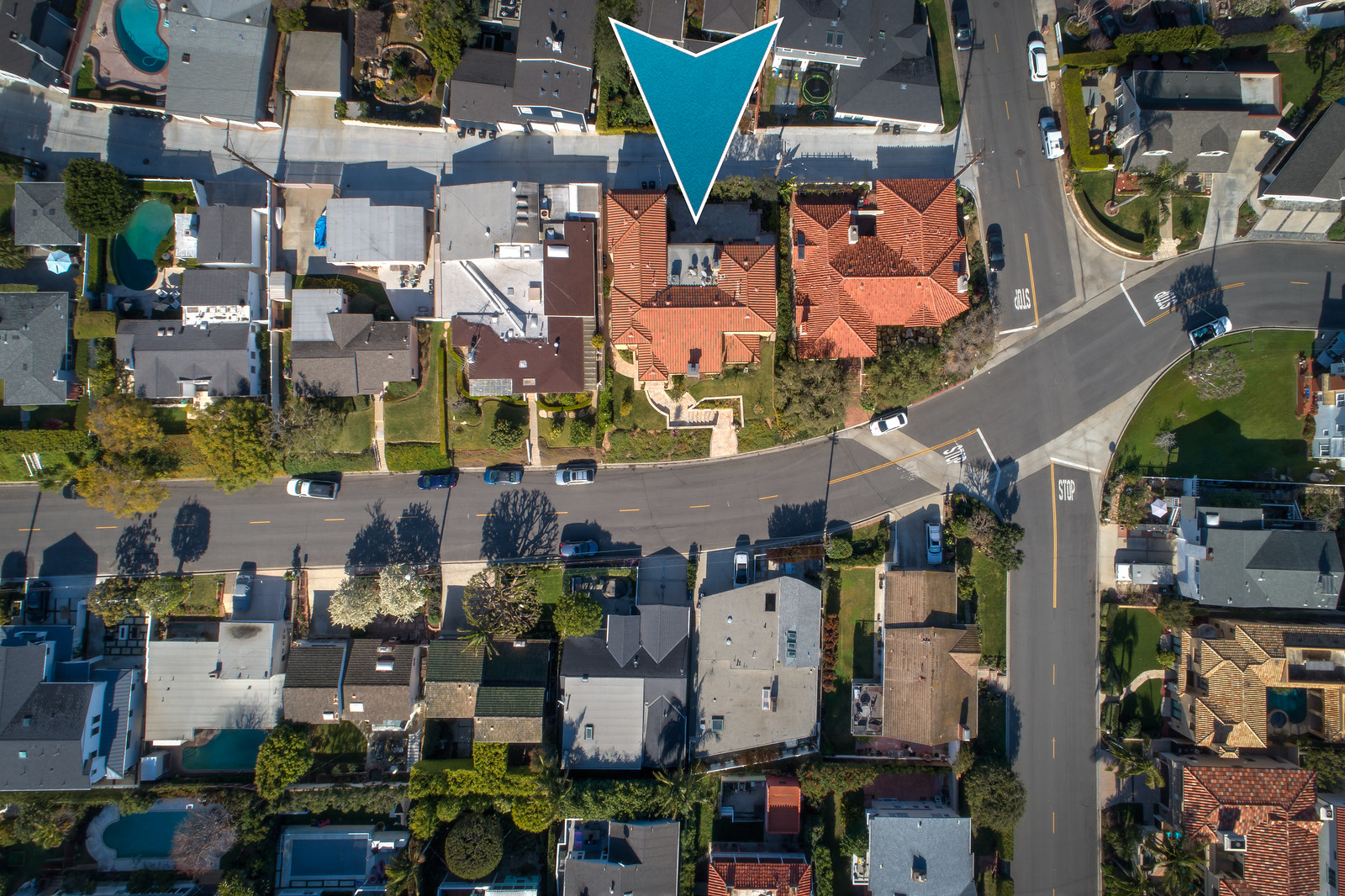This aerial photograph showcases a suburban housing area with numerous detached homes. In the center-top of the image, a blue arrow points towards a specific property, notable for its red roof. A central road traverses horizontally through the middle of the image, curving slightly upward to the right. On the upper side of this road, six distinctive houses line up side by side, each with unique driveway configurations and varied roof colors. Below the road, seven additional detached homes are visible, closely spaced yet individually distinct. Towards the right-hand side of the image, a vertical road intersects the main horizontal road, forming a crossroads. This well-organized layout of the suburb is captured in vibrant detail, highlighting the characteristics of each house and the overall structure of the neighborhood.